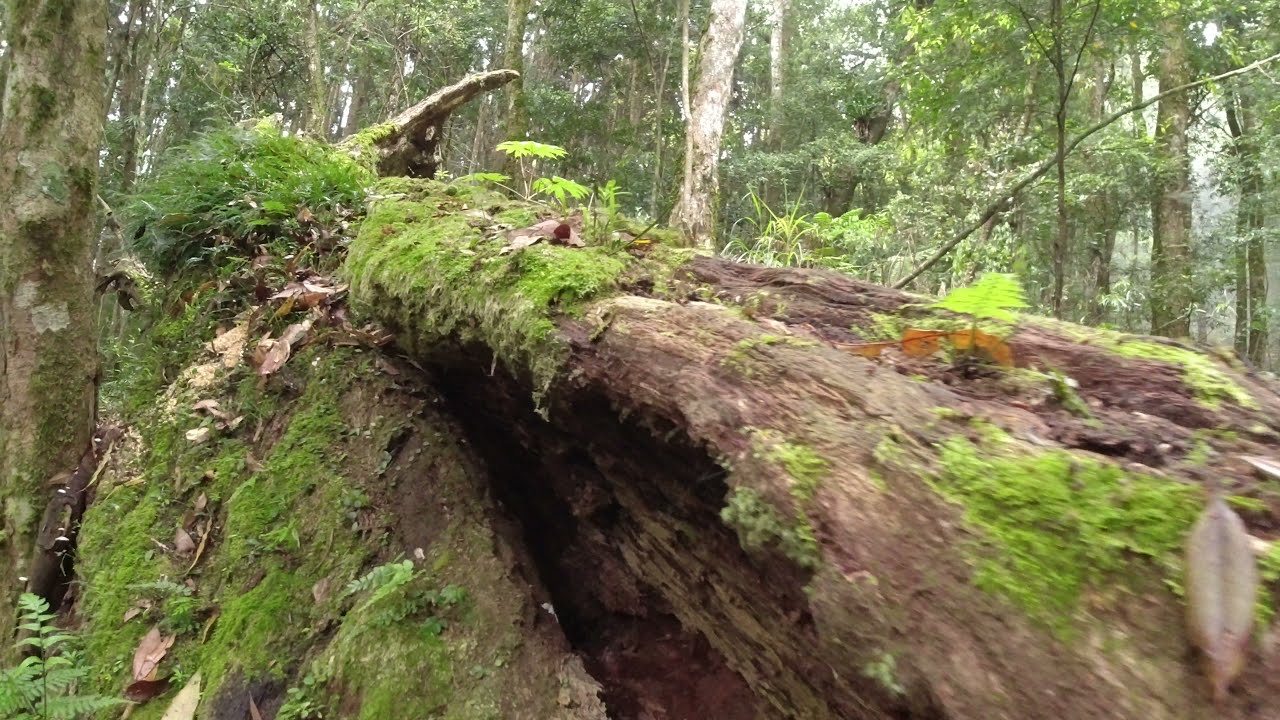The image showcases a close-up of a massive, decaying log or fallen tree trunk in a dense forest. Dominating the frame, the wood stretches diagonally from the upper left to the bottom and right sides, disappearing out of the picture. The log, which may have been uprooted or split by lightning, is covered in patches of bright green moss and dotted with dried leaves. Fluffy, grass-like plants and other vegetation sprout from the upper left corner of the log, while small ferns peek out from the forest floor on the lower left. Behind the giant log, a thick forest of tall trees with moss-covered trunks and dense green foliage fills the background, creating a rich, verdant backdrop. The scene captures the serene and ancient feel of this woodland area, highlighting the natural process of decay and regrowth.